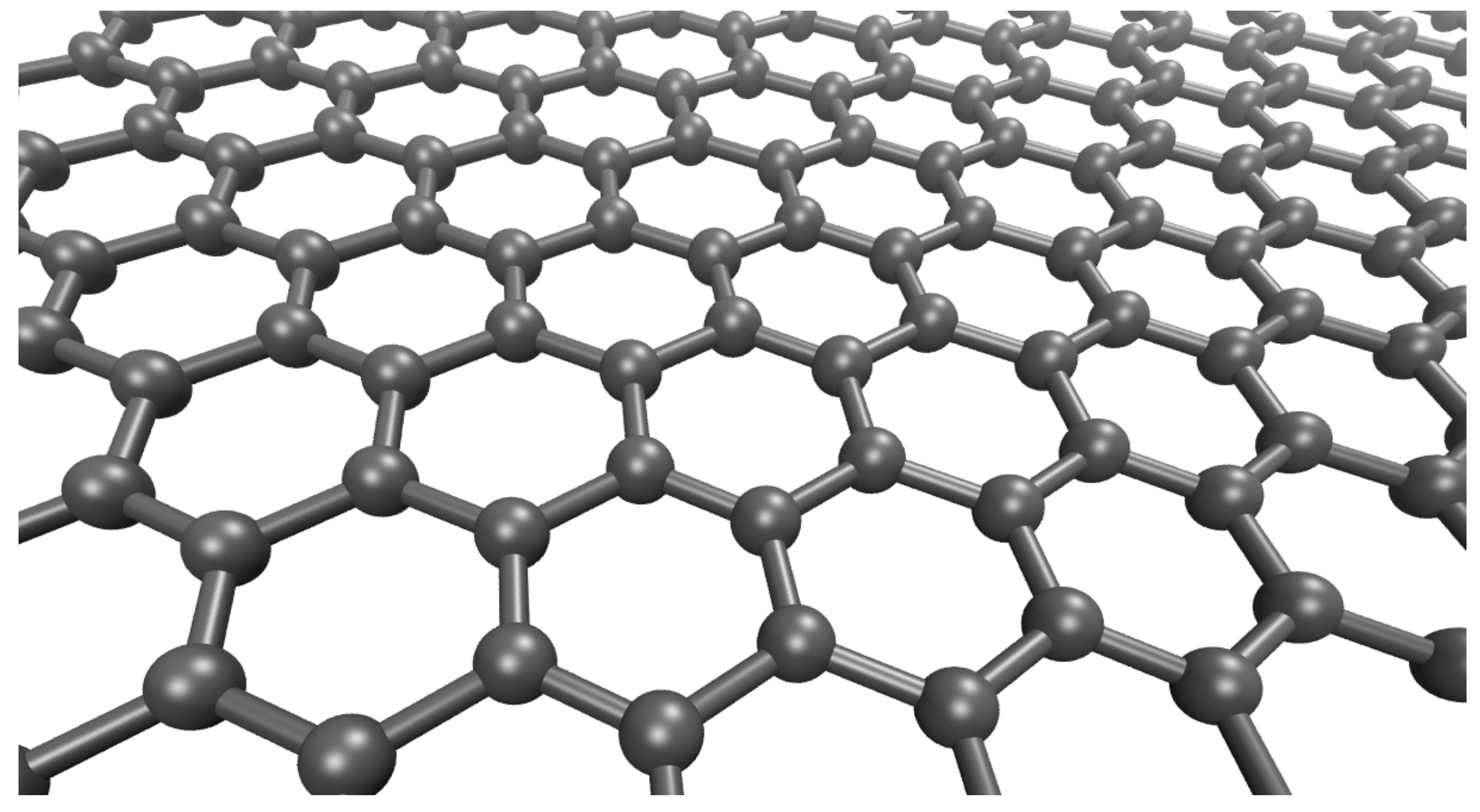The image depicts a detailed, digitally-rendered lattice structure set against a stark white background. It features a repeated pattern of hexagonal shapes constructed from dark gray or black tubes connecting shiny, reflective spheres at each of the six corners. These hexagonal units, visually interpreted as molecular structures, seamlessly connect to each other, creating a cohesive, expansive network that appears to recede into the distance, adding a sense of depth. The image, devoid of borders, text, people, or animals, focuses entirely on this intricate, scientific-like arrangement, emphasizing the symmetry and interconnectedness of the hexagonal lattice.